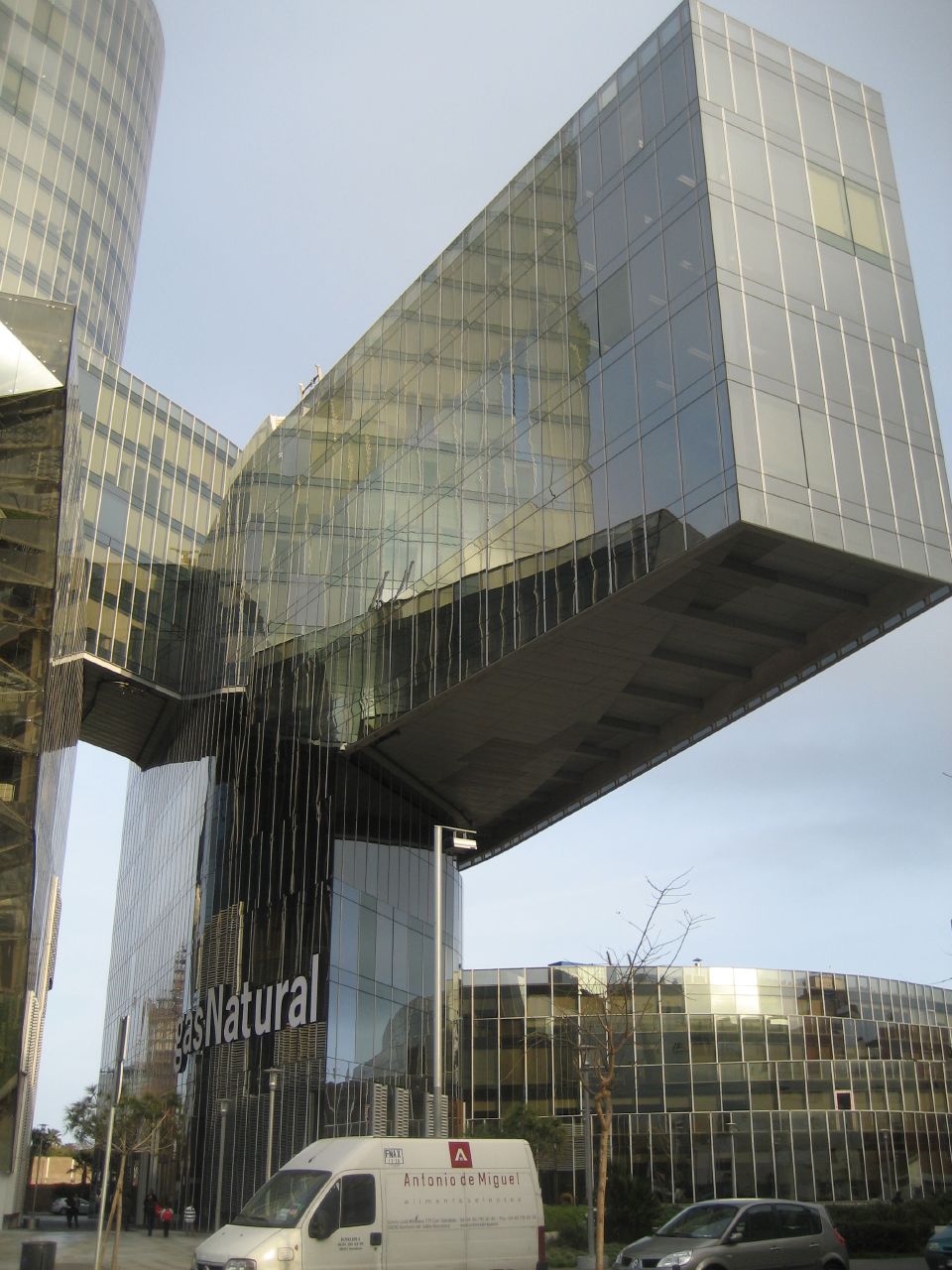This full-color daytime photograph, seemingly taken in a bustling city, showcases a remarkably unique architectural design. Dominating the center of the image is a large, modern building, predominantly made of glass, with the words “Gas Natural” prominently displayed on its façade. The innovative structure features dramatic sections jutting out horizontally from its vertical framework, creating an eye-catching silhouette against the blue sky. In the foreground, a white van with red lettering reading "Antonio de Miguel" is parked on the concrete walkway, alongside several other vehicles. Adjacent to the van is a lamppost and two small trees—one bare and the other with leaves. The ground surfaces include both the sidewalk and the nearby road, further emphasizing the urban setting. The scene is a vivid mix of colors including light blue, gray, tan, brown, white, red, orange, and green, highlighting both the natural and built environment in this intriguing composition.